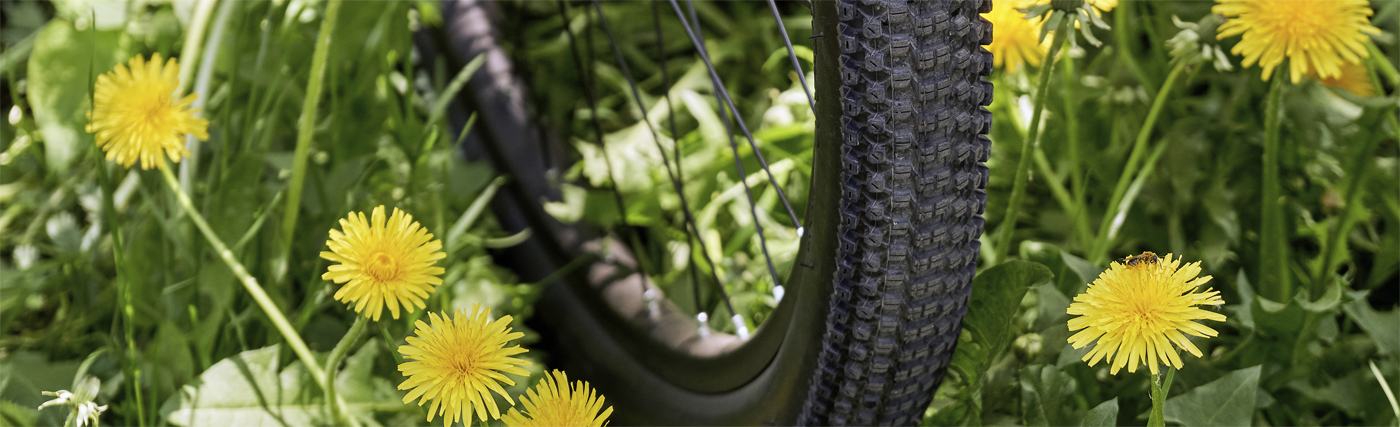This is an up-close photograph taken from ground level, capturing the bottom third of a thick, black mountain bike tire with deep treads and black spokes interspersed with silver. The tire is moving through a lush field brimming with yellow daffodils. The image reveals seven prominent daffodils—four on the left and three on the right—all with multiple petals and yellow centers. The scene is teeming with green and yellow hues, complemented by various leaves, grass, and weeds visible around the tire. Notably, a brown bug perches on one of the flowers on the right. Additionally, a white object, possibly an abandoned face mask, lies on the ground to the left of the tire, adding an intriguing element to the natural setting. The background is intentionally blurred, emphasizing the vivid foreground elements and providing a sense of motion as if the tire is riding through the field.